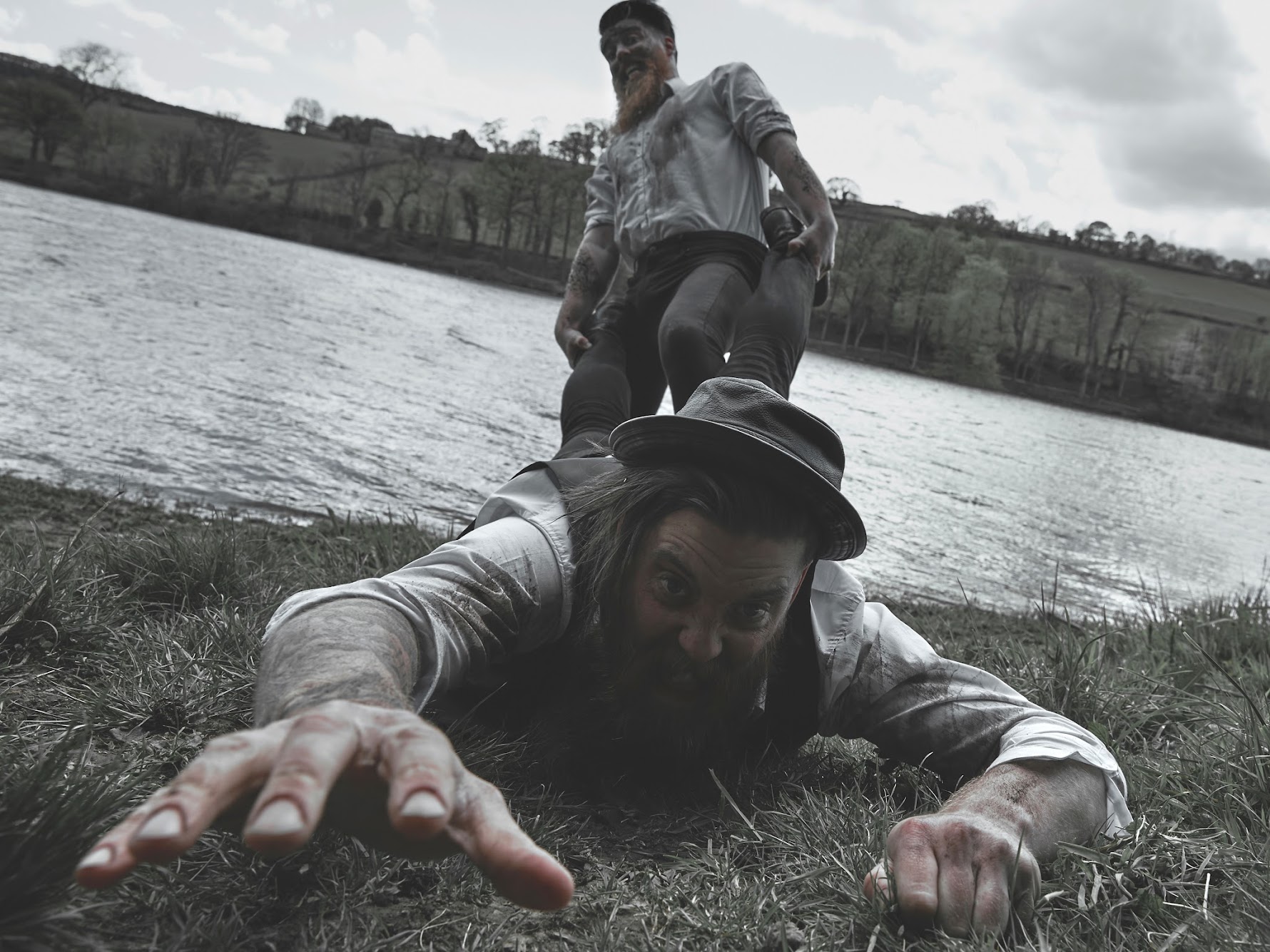The image depicts a humorous scene of two men dressed in 18th-century attire by the side of a large body of water. The man in the foreground is trying his best to avoid being dragged into the lake (or river), his chest against the ground, his hands desperately grasping at the grass but finding no purchase. Both men are wearing white, long-sleeved blouses with vests and hats, adding to the historical costume. The man doing the dragging has a distinct orange-colored beard with hints of brown, and a determined look on his face. The photo itself has a stylized, partially black-and-white aesthetic with muted colors, particularly emphasizing the hands. The grassy background and expansive water body create a dramatic yet playful backdrop for this scene that captures the lighthearted struggle between the two characters. They both have expressive, almost comical looks, clearly indicating the playful nature of the moment.